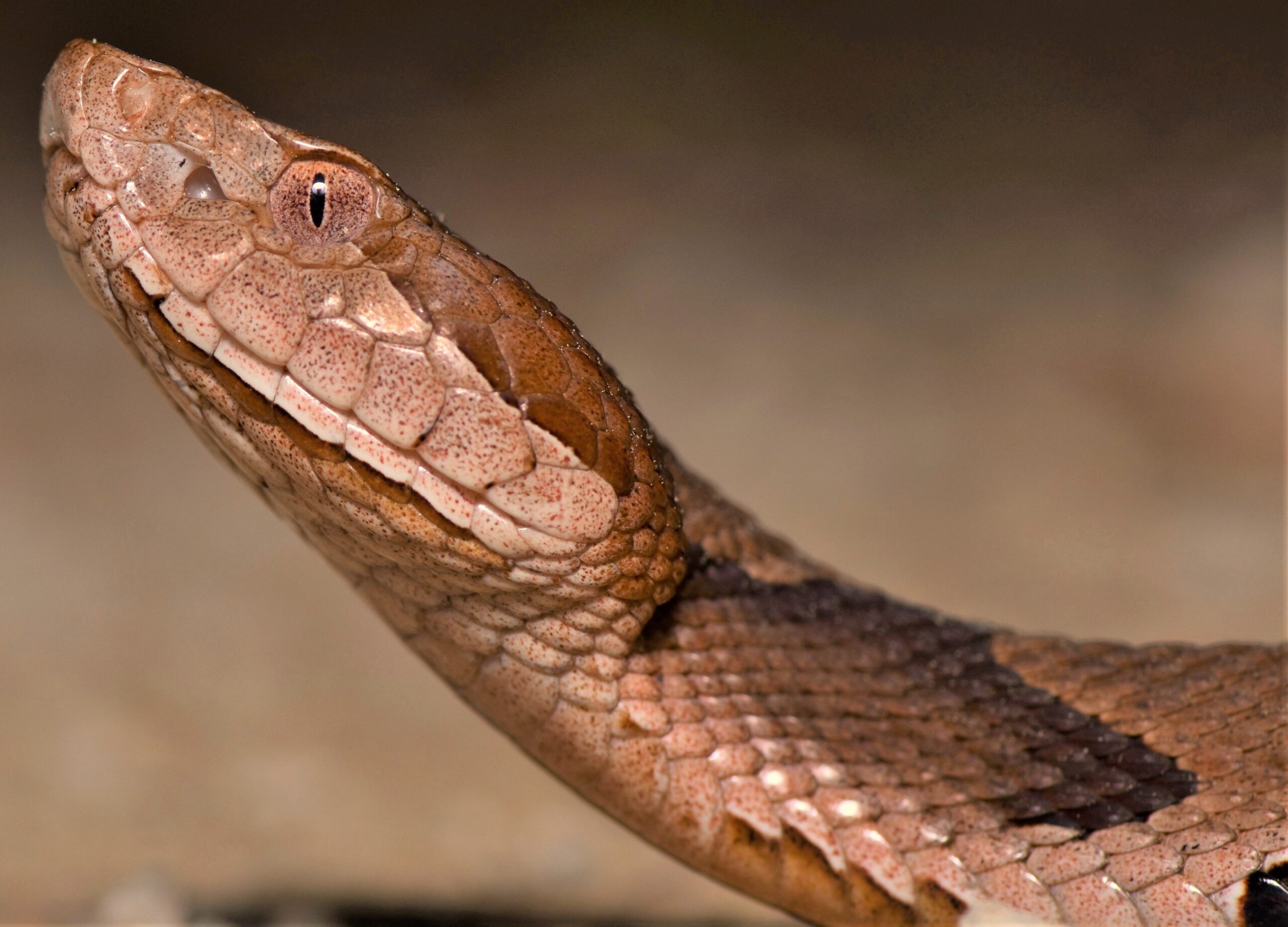This is an extremely up-close photograph of a snake's head and the upper portion of its body, capturing it from a side profile. The snake's scales exhibit a mesmerizing array of colors, predominantly dark brown, tan, and light tan, with a golden hue. There are also noticeable black streaks and speckled patterns, particularly under the eyes, and a distinctive copper coloring that suggests it could be a copperhead. The snake’s brownish-tannish eye, detailed with dark red specks, is clearly visible in this tightly focused shot. The background is blurred and fades into a beige color, ensuring that the entire attention remains on the intricate details of the snake’s scales and patterns.